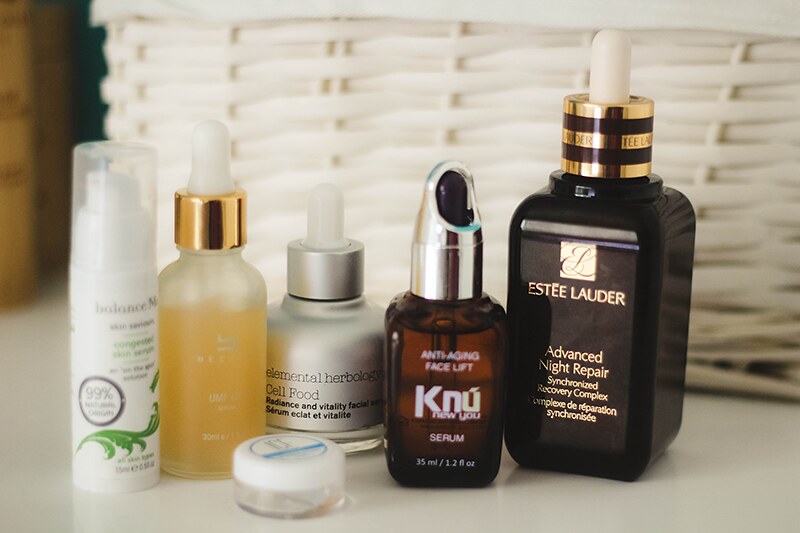The image features a woven basket placed at the back, filled primarily with white leaves. The tabletop is white, adding a crisp contrast to the assortment of containers arranged in front. On the far left, there's a white tube with a clear top and some text, next to which green leaves are visible, defining less than 99%. Next to it is a clear bottle containing yellow liquid, equipped with a dropper. Further to the right, there's a silver container labeled "Cell Food" in a small jar, followed by a clear brown bottle labeled anti-aging facelift serum with a silver top. Another dark-labeled container displays a prominent symbol reading "E Lauder," with a bronze and black striped design extending to the top. The container is topped with a white rubber dropper handle, labeled "Advanced Night Repair, Synchronized Recovery Complex." Various shadows add depth and dimension to the scene.